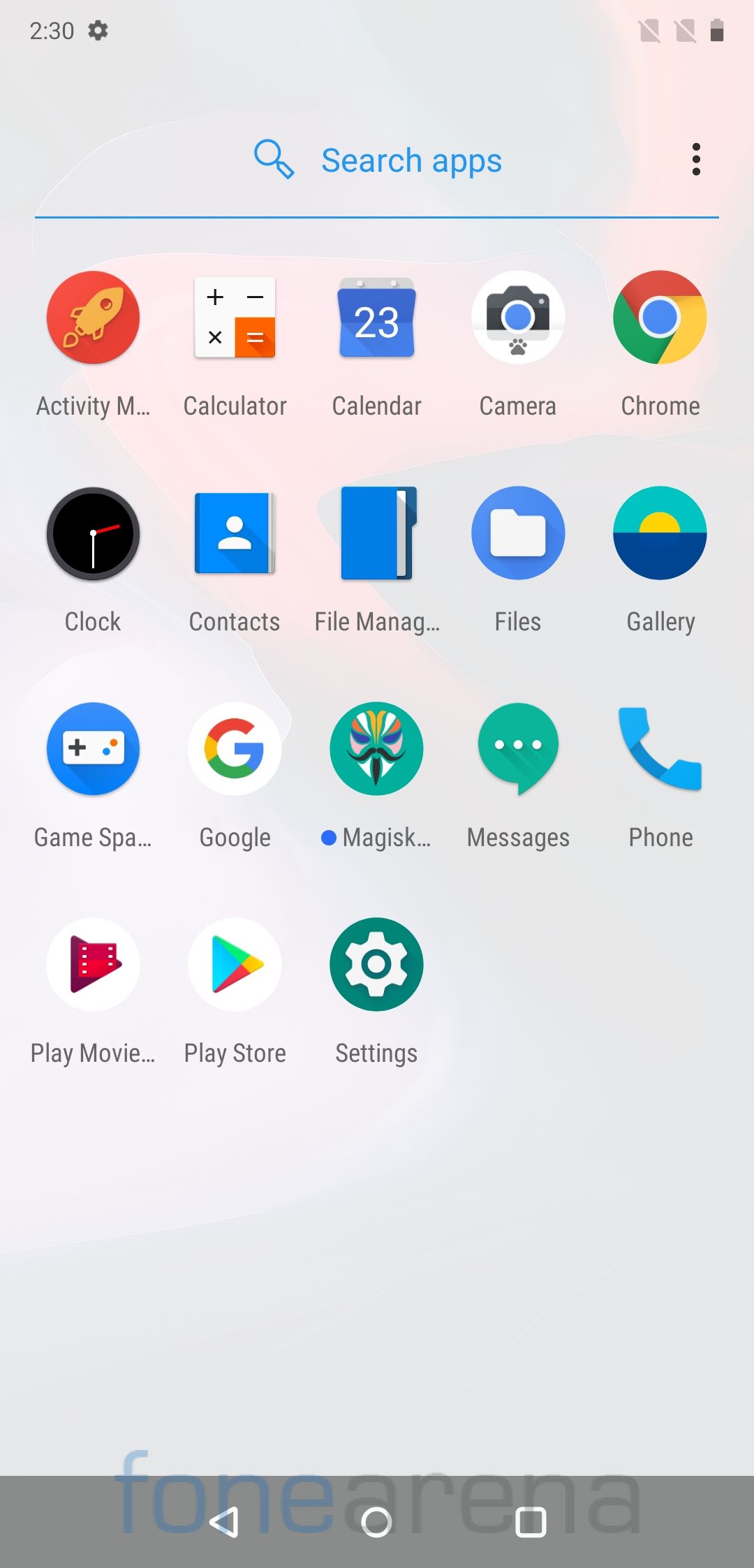The image displays a screenshot of an Android phone's search screen for apps. The screenshot was taken at 2:30, though it is unclear whether it's a.m. or p.m. The battery level, located in the upper right corner, is approximately 60% full.

At the top of the screen, there is a search bar with the text "Search apps" in blue, though no specific search query has been entered. Below the search bar, several app icons are displayed in four rows. The first three rows contain five app icons each, while the fourth row contains three. 

The visible app icons include:

- An activity monitor
- Calculator
- Calendar
- Camera
- Chrome
- Clock
- Contacts
- File Manager
- Files
- Gallery
- Game
- An app labeled "spa" followed by an ellipsis suggesting it is abbreviated (S-P-A…)
- Google
- Magisk (displayed as "Magisk…", indicating truncation)
- Messages
- Phone
- Play Movies
- Play Store
- Settings

At the bottom of the screen, there is an apparent branding or watermark that reads "FoneArena," with "Fone" in blue and "Arena" in gray.